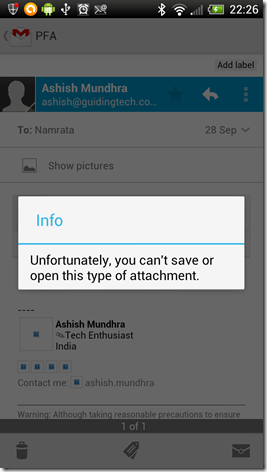Here's a detailed and cleaned-up caption for the image described:

---

The image is a mobile screenshot taken from an Android device, which could be either a phone or a tablet. The notification bar at the top displays several icons including a shield with a red notification, an orange circle with a white line through it, a small Android logo, a Share or USB icon, an alarm symbol, and an icon that resembles a screw with a square on its side. The device's Bluetooth is switched on, it is connected to Wi-Fi with three out of four bars, but has a poor cellular signal with only one out of five or six bars. The battery level is about 75%, and the time is 22:26.

In the background, the Gmail app is open. The email is from Ashish Mundra (ashish@guidingtech.co) and is addressed to Namrata, dated September 28th. The interface shows a white arrow to go back and three dots for more options. There is a prompt asking whether to show pictures, alongside a pop-up error message stating, "Unfortunately, you can't save or open this type of attachment."

Below the error message, Ashish Mundra's name is repeated along with the title "Tech Enthusiast India." However, icons for various contact methods are not loading properly, displaying blue question marks instead. A disclaimer starts to appear, reading, "Warning, although taking reasonable precautions to ensure," but is cut off and incomplete. The email indicates it is the first and only message in the thread.

At the bottom of the screen, there are icons for trash (delete), checklist, and mail, suggesting the user might be attempting to send an email but is unable to attach a specific file.